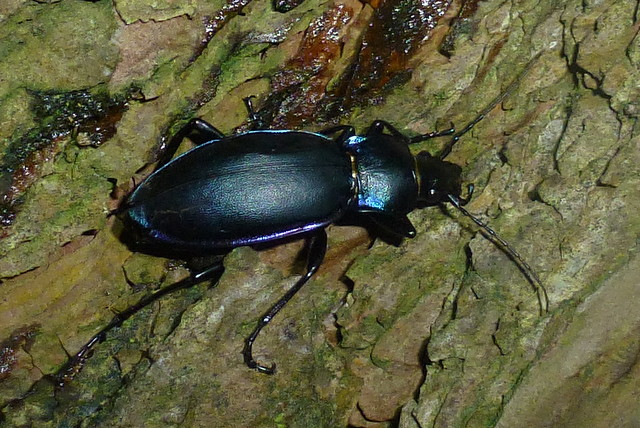This detailed image showcases a rather large black beetle perched on a piece of sticky, wet tree bark. The beetle's body, exhibiting a glossy sheen, reveals iridescent hues of blue and purple along its edges, which might be due to the reflection of light. Its distinct anatomy includes three visible body segments: a small head with two long feelers or antennas on each side, an intermediate slender section, and a long, almond-shaped posterior. The beetle's six pointy legs are prominently seen clutching onto the bark, which appears to be saturated with sticky tree sap, giving it a shiny and somewhat reddish-brown appearance. The surface the beetle is on could be varied hues of green and grey, indicating a natural setting, possibly enhanced by the moisture from the sap.